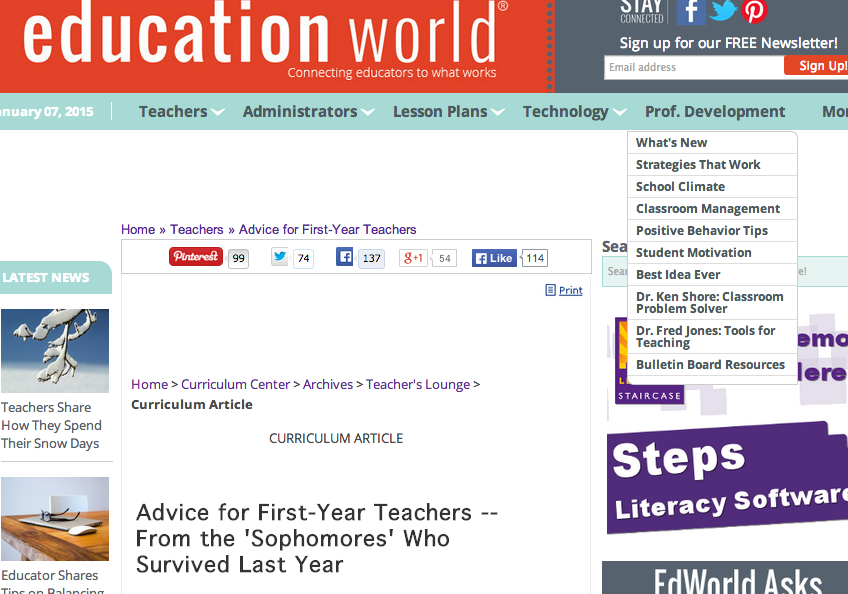In the top left corner of the image, there is a red box containing large, white, lowercase letters that spell out "Education World." Directly below this, in smaller text, it reads, "Connect an educator to what works." Underneath, there is further text displaying the date, "January 07, 2015," followed by a list of keywords: "teachers, administrators, lesson plans, technology, professional development, what's new, strategies that work, school climate, classroom management, positive behavior tips, student motivation, best idea ever, Dr. Ken Shore classroom problem solver, Dr. Fred Joan tool for teaching, bulletin board resources."

In the center of the image, there is a section labeled "Home" and "Curriculum Center." Adjacent to this, an archive labeled "Teachers Lounge" can be found. In this area, the text reads, "Curriculum article: Advice for a first year teacher from the sophomores who survived last year." Further down, an image of a tree branch with snow on it appears, along with the text "Latest News: Teachers share how they spend their snow days." At the bottom, the words "Steps Literacy Software" are displayed.